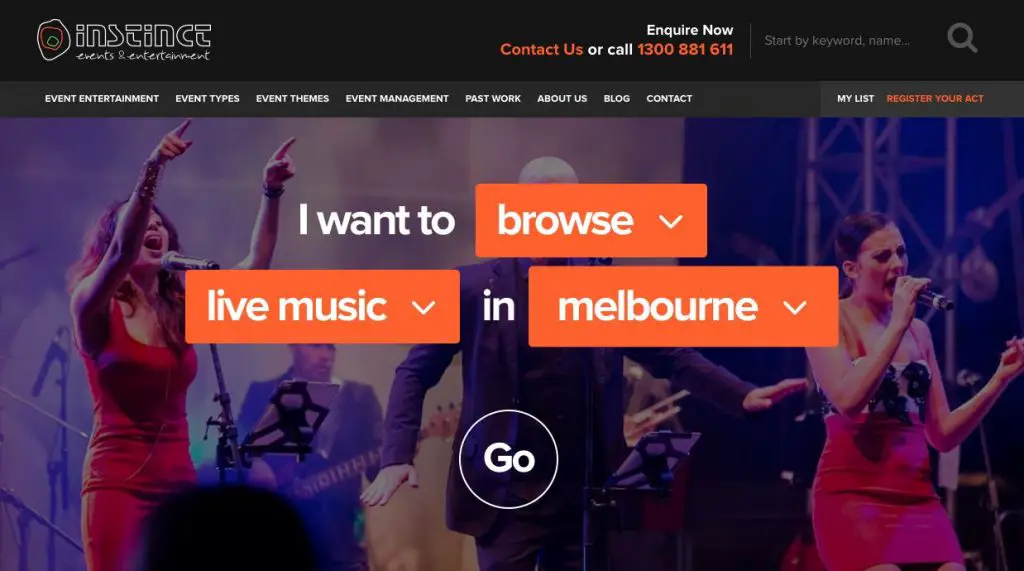The screen capture showcases the landing page of a website likely named "Instin.ce." The webpage appears to be dedicated to music, specifically live music events. Central on the page, there is a prominent text overlay featuring three dropdown menus. The first dropdown reads, "I want to browse," with the word "browse" contained within an orange rectangle. Directly below it, another orange-rectangled dropdown states "live music," followed by a third dropdown with the location "Melbourne," also in an orange rectangle. Each orange rectangle has an arrow pointing downward, indicating they are interactive dropdown menus. 

Below these dropdown menus, there is a circular button with the word "Go" in white font. The background of the page features an image of people performing on a stage, suggestive of a live music scene. 

In the upper right corner, the page provides contact information, including options to "Inquire now," "Contact us," or call 1-300-881-611. The upper navigation ribbon includes tabs for different sections of the website: Event Entertainment, Event Types, Event Themes, Event Management, Past Work, About Us, Blog, and Contact.

The detailed layout and elements suggest that this website allows users to browse and access information about live music events based on specific parameters such as type and location, particularly focused on Melbourne.